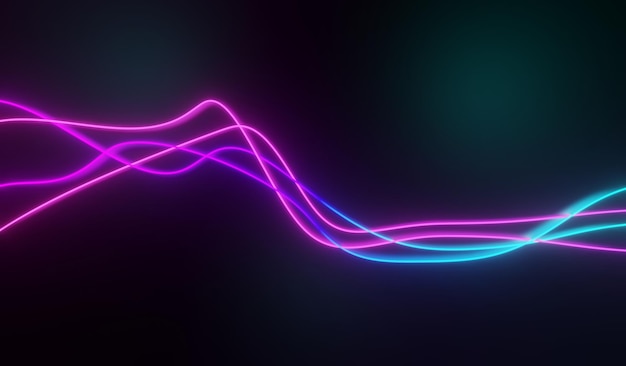The image depicts a striking neon light display against a solid black background. Four undulating lines, reminiscent of computer-generated visuals synced with music, horizontally traverse the frame from left to right. These interwoven neon tubings start with a deep purple hue. Two of the lines maintain this purple color throughout their journey, while the other two lines gradually transition into a vibrant blue, eventually shifting to a very light, almost greenish-blue as they reach the right side. Accentuating the visual are faint blue glows in the background, one notably on the upper right and a smaller one on the upper left, adding a subtle depth and mystique to the composition. The overall scene blurs slightly into gray in some spots, enhancing the dynamic and almost ethereal quality of the lights against the otherwise solid black backdrop.